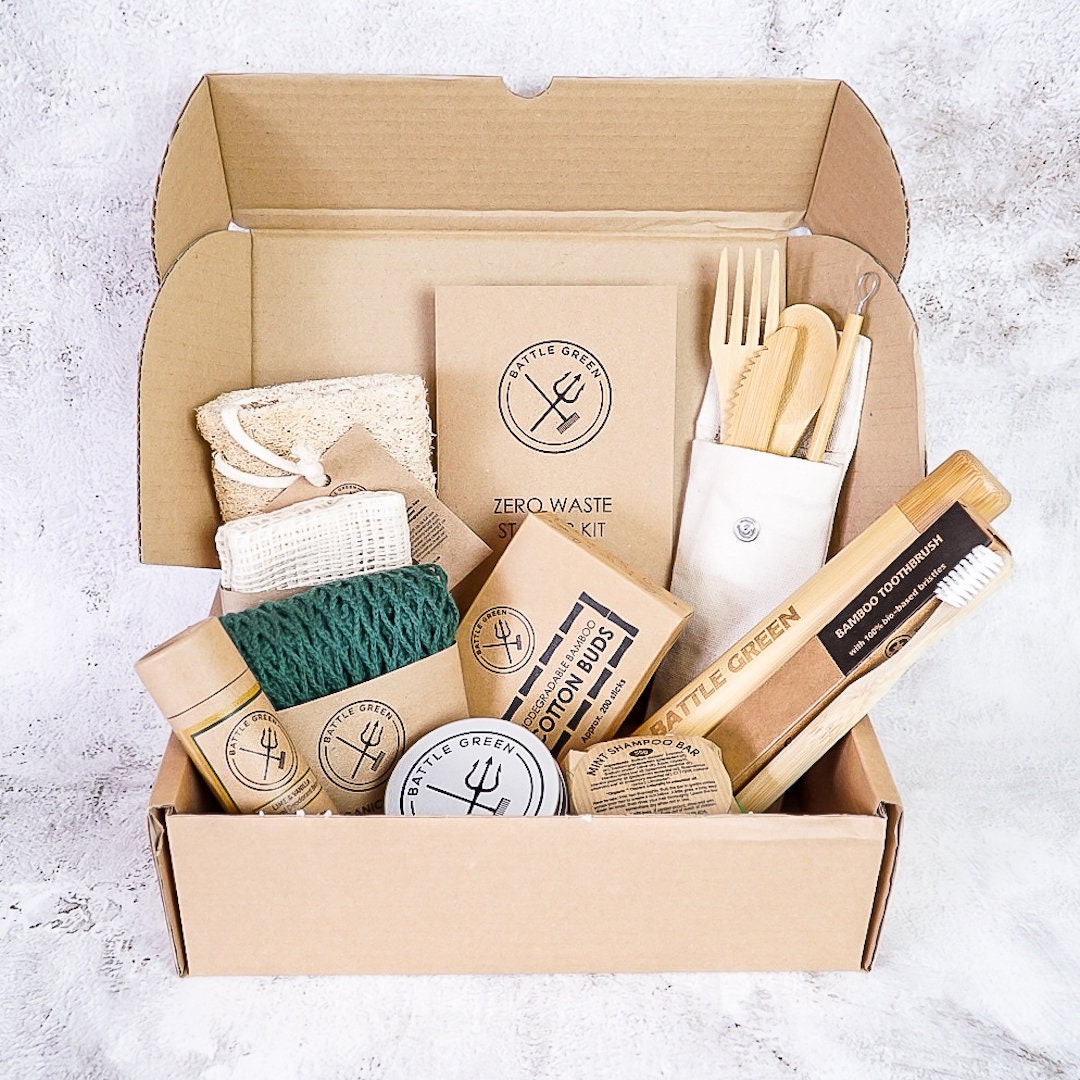The image features a monthly subscription box available for purchase, curated by the company Battle Green. The company's logo is prominently displayed, consisting of a circle with a trident pointing toward the upper right corner and a mop angled toward the lower right corner, both crossed.

Inside the box is a carefully arranged assortment of eco-friendly products, emphasizing the brand's commitment to sustainability. The centerpiece of the package is a label that reads "Zero Waste Starter Kit." To the right, a set of wooden utensils, including a fork, spoon, and knife, are neatly placed, indicative of their reusable nature. 

In the foreground, another wooden tool labeled with "Battle Green" is visible, signifying the company's branding on practical items. Among the products included, you can also find a bamboo toothbrush, a refreshing mint shampoo bar, biodegradable cotton buds, and eco-friendly sponges suitable for use in the shower. These items collectively aim to promote a zero-waste lifestyle and provide users with sustainable options for daily hygiene and grooming.